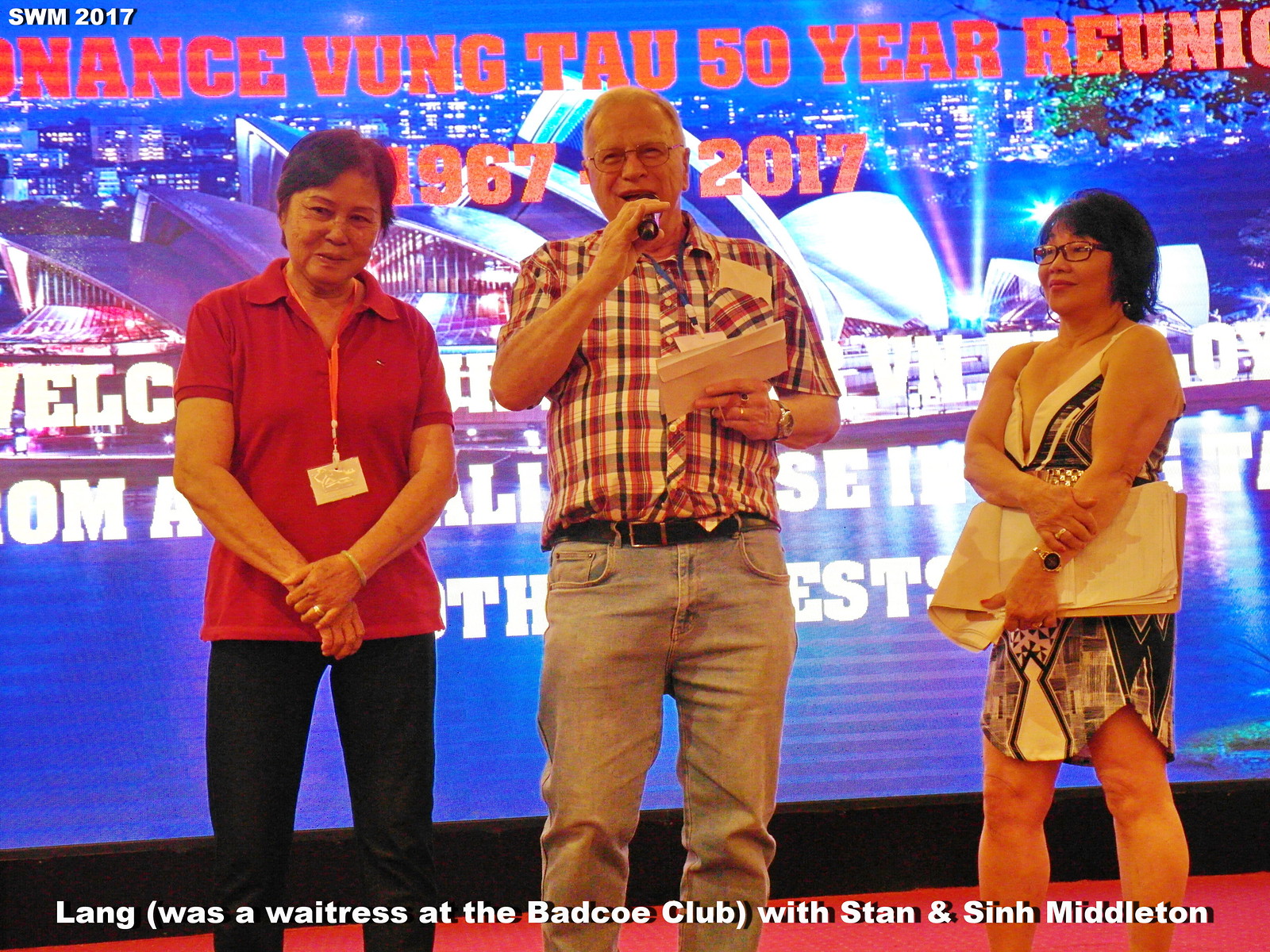This detailed photograph captures three individuals on a stage in front of a large banner that reads, "Nance Vung Tau 50-Year Reunion 1967-2017." The banner features an image that resembles the Sydney Opera House, positioned against a body of water, with additional, smaller text that is unclear. 

On the left stands a woman with short black hair, wearing a red polo shirt and black pants. She has a lanyard around her neck, and her arms are folded as she looks down with a smile. 

In the center is a man sporting glasses and exhibiting a balding head. He is speaking into a microphone, holding it in one hand, and in the other, he has an envelope or card, possibly indicating he is about to present an award or make an announcement. He is dressed in a checkered short-sleeved shirt paired with pale blue jeans.

On the right is another woman with short black hair and glasses. Unlike the woman on the left, she does not have a lanyard around her neck. She holds a sketch pad or clipboard and stands with her arms folded, looking straight ahead. 

Below them, there is white text that reads, "(was a waitress at the Bad Co. Club) with Stan Middleton."